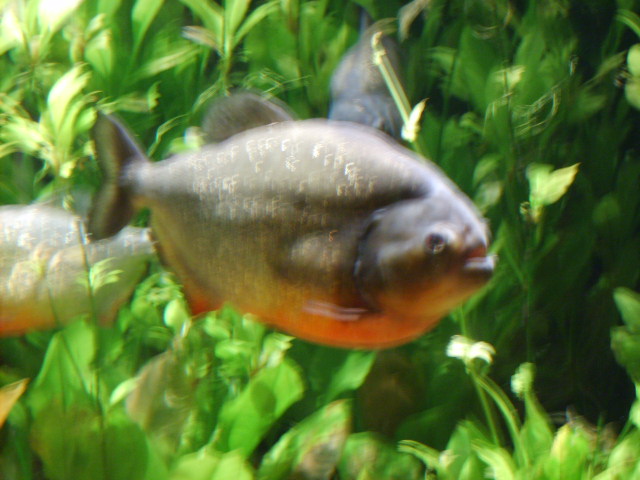The image captures a close-up, slightly out-of-focus scene within an aquarium, featuring three fish amid lush, green seaweed and coral. The central fish, somewhat large and round with a distinctive coloration of gray on top, white in the center, and an orange-red underbelly, is swimming briskly from left to right, possibly startled by the camera's proximity. Its small tail fin, rounded dorsal fin, and small mouth are noticeable, along with its solitary round eye. In the backdrop, amidst the shiny, bright green foliage which provides ample camouflage, a second fish emerges beneath the algae on the far right, while a third fish is swimming from right to left. The vibrant greenery indicates a well-maintained environment, adding to the overall bright and appealing aesthetic of the scene.